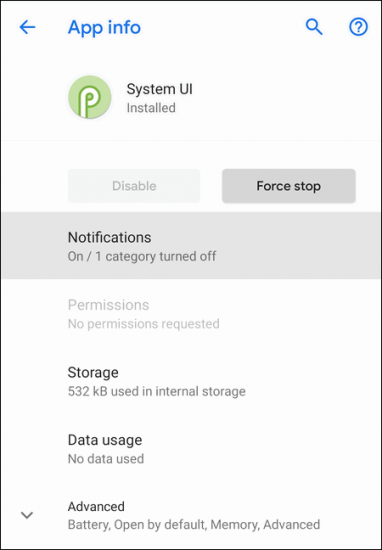In the image, we observe a screenshot of an Android phone's app settings interface.

At the top left, a light bluish arrow points to the left, suggesting a navigation option to go back. Adjacent to this arrow, in the same light blue text, is the label "App info."

In the top right corner, a blue circle contains a question mark, likely for help or additional information. To its left, a blue magnifying glass icon points diagonally towards the top left, probably for searching within the app settings.

Centrally aligned beneath these elements is a light green circular logo with a white letter "P" in its center, representing the app icon. Next to this logo, the app name "System UI" is written in black text, and directly below it, the status "Installed" appears in a grayish color.

Just below these details are two rectangular buttons: "Disable" on the left and "Force stop" on the right.

In the middle of the image, a large gray rectangular section spans the width of the screen, displaying the text "Notifications: On / 1 category turned off."

Further down, the following information is listed:

- "Permissions: No permissions requested"
- "Storage: 532 KB used"
- "Data usage"
- "Advanced"

This detailed visual layout provides comprehensive settings and information about the System UI app on an Android device.